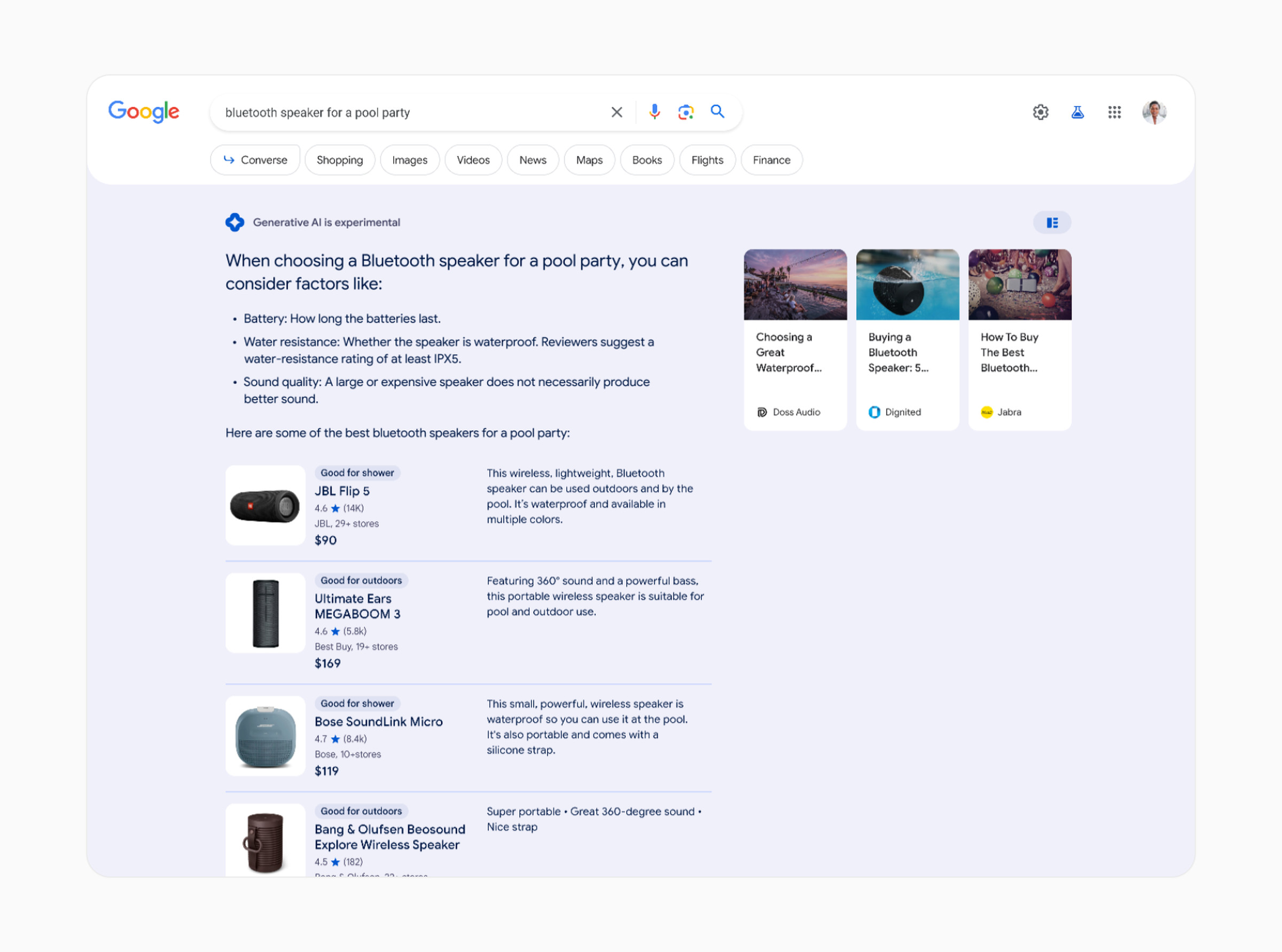The image is a detailed screenshot of a Google search page. In the top-left corner, the Google logo is displayed in its classic blue, red, yellow, and green colors. At the center of the page is the search box, in which the text "Bluetooth speaker for a pool party" has been entered. Adjacent to the search box, a small 'X' icon is visible, along with a blue microphone icon and a blue magnifying glass icon.

To the right of the search box, there is a thumbnail image featuring a man dressed in a white jacket. Below the search query results, several images of Bluetooth speakers are displayed. 

The first image features a black speaker sporting a small red dot, identified as the JBL Flip 5. Beside this speaker, additional information is provided, highlighting its 4.6-star rating and a price of $90. The description notes that this wireless, lightweight Bluetooth speaker is suitable for outdoor use and is waterproof. It is also available in multiple colors.

Another speaker is shown in the next image, a gray device labeled Bose SoundLink Micro, priced at $119. Below this, three smaller rectangles display various images; notably, one depicts a speaker being submerged underwater, emphasizing its waterproof capability.